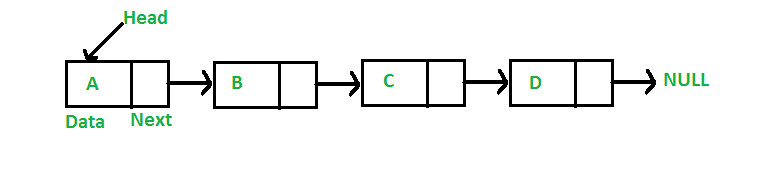This image is a digitally created, landscape-oriented illustration with a clean, white background. Four horizontally aligned rectangles, each with a black outline, are spaced evenly with about an inch between them. Each rectangle is divided into two parts: on the left, two-thirds of the space is filled with white, and on the right, a vertical black line separates the remaining one-third, which is also filled with white.

In the first rectangle, the left side features a green letter "A" with the word "DATA" written in green below this section. On the right side of the first rectangle, the word "NEXT" appears in green under its corresponding section. Above the green letter "A," there is a downward-pointing arrow accompanied by the green text "HEAD."

Each subsequent rectangle follows a similar structure. The second rectangle has the green letter "B" on the left side with no additional text below. The third rectangle exhibits the green letter "C" in the same position, while the fourth rectangle displays the green letter "D."

Between each pair of adjacent rectangles, a rightward-pointing arrow connects them, indicating a flow or sequence from one to the next. Finally, to the far right of the fourth rectangle, a rightward arrow extends toward the word "NULL" written in green, which signifies the end of the sequence.

The image effectively represents a sequence or process flow, starting with "A" and ending with "NULL," with clear navigation cues in the form of arrows.